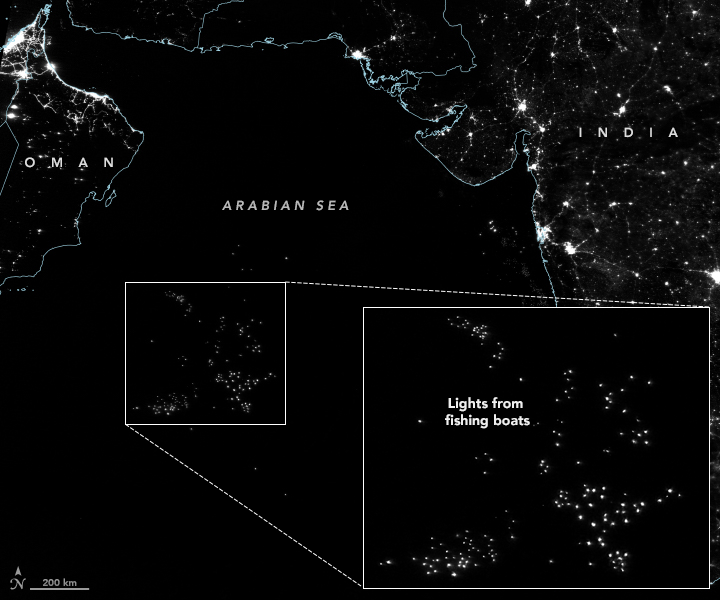This image is a black-and-white satellite photo with a subtle blue tinge highlighting the borders, depicting a nighttime view over the Arabian Sea. On the left, the country of Oman is marked, and to the right, India is labeled. Both countries have outlines in a dark blue color. The sea itself is labeled "Arabian Sea." 

The main focus of the image is the contrast between dark and light areas. Predominantly dark, the image shows bright white dots and specks scattered across the Arabian Sea, which are identified as lights from fishing boats. These tiny lights are further zoomed in within an inset square that emphasizes their presence.

The coastlines of India and Oman are illuminated with larger, more concentrated splotches of light, representing city centers, while smaller lights dot the interior regions of both countries. This suggests a higher concentration of human activity along the shores. The borders and outlines created with a dark bluish hue clearly delineate the landmasses from the sea, visually framing the detailed distribution of nighttime lights in this region.